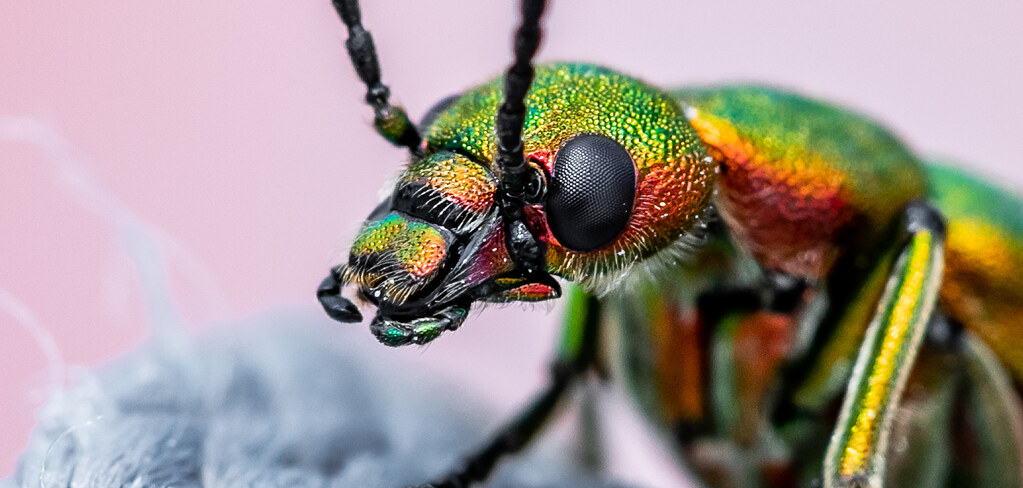This is an incredibly detailed close-up photograph of an insect, predominantly filling the right two-thirds of the frame. The insect's upper body is vividly captured, showcasing a large, textured black eye and two segmented black antennae flanking the eye. Its head and body exhibit iridescent shades of shiny green and yellow, with hints of red around its eyes and head, and a subtle coppery bronze sheen. Its mandibles and mouthparts are clearly defined. The insect appears to be standing on a grayish, fuzzy object, possibly resembling cotton or carpet fibers, situated towards the lower part of the image. The background features a pale lavender or pinkish hue, adding contrast to the insect's vibrant colors. The insect's body, apart from the head and upper torso, is blurred out, further emphasizing the detailed textures of its head and facial features.